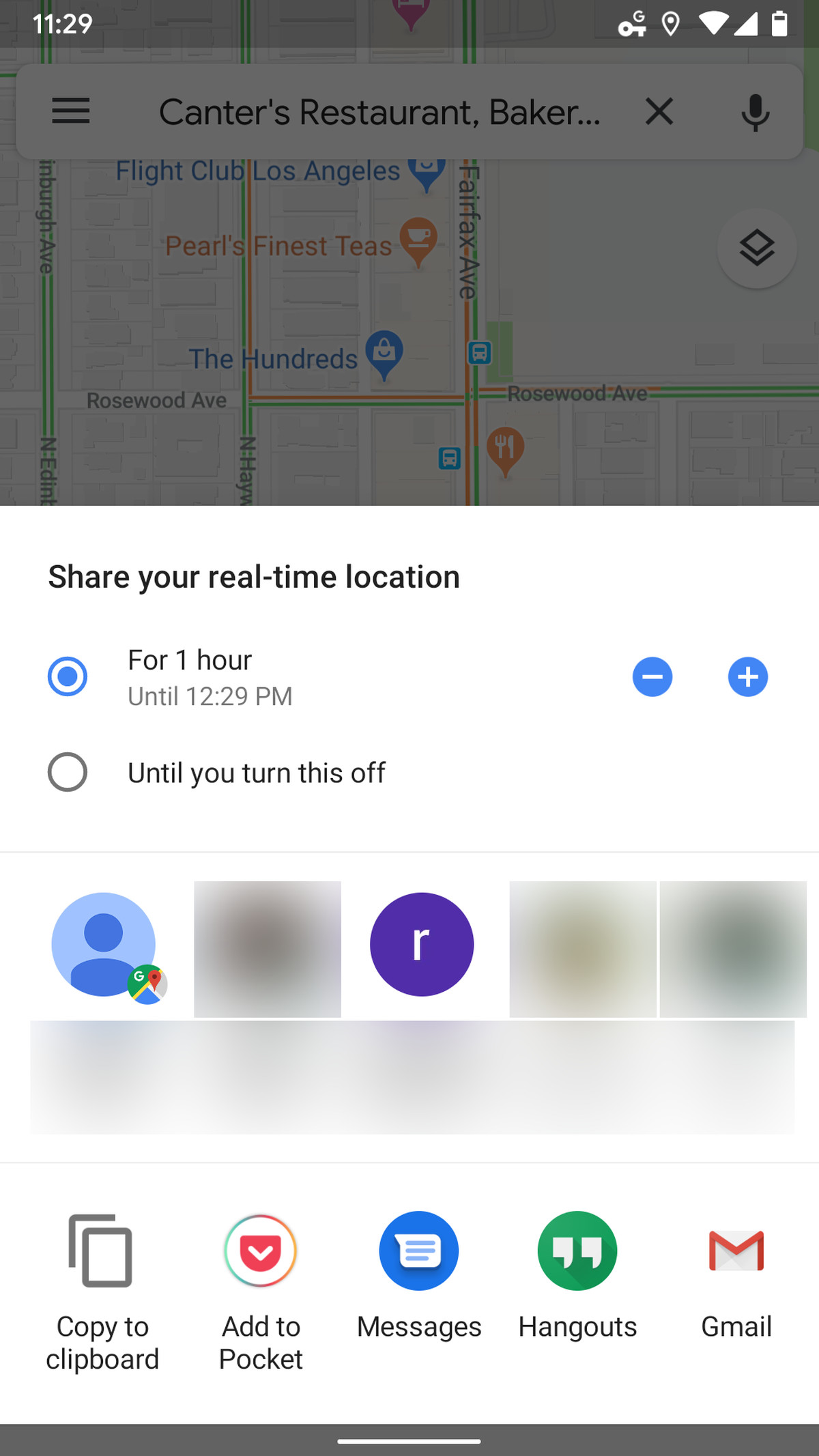This image features the Google Maps app interface, identifiable by its characteristic map design and familiar icons used for pinning locations. Notable icons visible include one for shopping and another believed to be for food. At the top of the screen is the signature white search bar with three lines indicating a dropdown menu on the left side. The search bar contains partial text reading "Cantor's Restaurant, Baker..." before it gets cut off. To the right of this text, there is a black 'X' for clearing the search field and a microphone icon for voice search.

Moving into the map view, the upper right-hand side features a white circular icon with a slanted square inside it, along with a border wrapping around one corner of the square. Towards the bottom center of the screen, a pop-up appears with a white background and bold black text that reads, "Share your real-time location." Below this message, there are two selectable checkboxes. The first box, which is checked and highlighted in blue, reads "For one hour," with further details below in small gray text stating "Until 12:29 PM." The second checkbox says "Until you turn this off." To the right of these options, there are two blue circles with white symbols: a minus sign in one and a plus sign in the other, likely for adjusting the time duration.

Underneath these options, several user icons are displayed. Although most are blurred out, the first one is visible, featuring a blue background with a user silhouette. Another discernible icon has a dark purple background with a white lowercase 'r'. This detailed description encapsulates the main elements and layout of the Google Maps app as presented in the image.